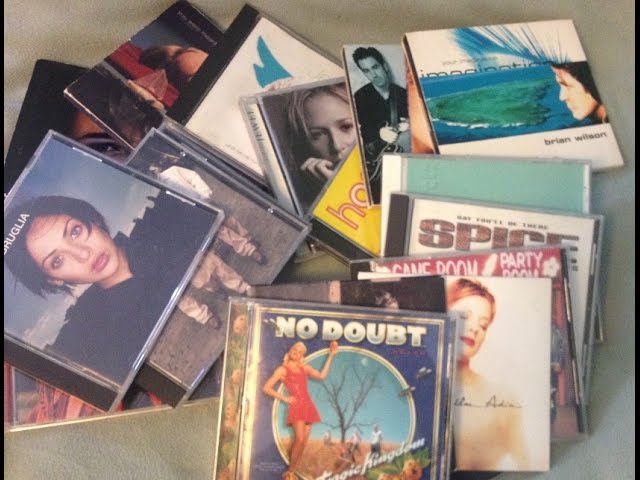The image depicts an eclectic assortment of colorful CDs scattered on a white table surface. Among these are clearly visible albums such as No Doubt, featuring a cheerful young blonde woman with her hand on her hip, possibly holding a soda, and Spice by the Spice Girls. Another identifiable album is from Christina Aguilera. They are casually fanned out, some CDs lying atop others, creating a vibrant, collage-like display. This collection, predominantly consisting of pop music albums from the 90s, includes around 18 CDs, with some obscured beneath others. The transparent acrylic cases reveal various album artworks, adding to the lively mosaic of 90s musical nostalgia. The background is a simple plain gray, allowing the colorful album covers to stand out prominently.